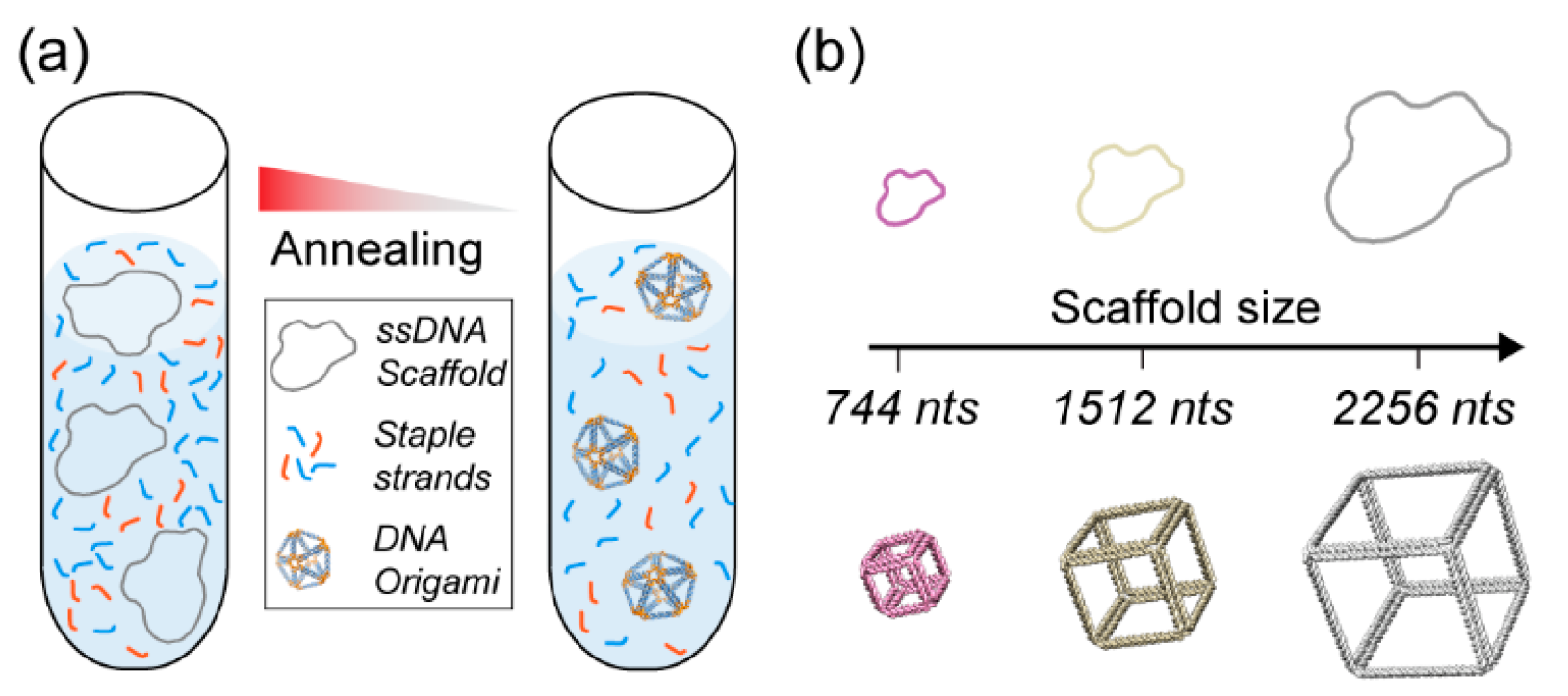The image consists of two labeled sections, A and B, both containing detailed scientific illustrations related to DNA. Section A features two test tubes in what appears to be a liquid environment, displaying content labels such as ssDNA scaffold, staple strands, and DNA origami. Above the test tubes, a chart titled "annealing" shows a red-to-gray gradient triangle. Below this are depictions for ssDNA scaffold (blobby outline shape), staple strands (five squiggly lines, three blue, two red), and DNA origami (a multi-dimensional structure). These elements are visually represented in the test tubes: one mixes DNA scaffold and staple strands, while the other combines these components into a DNA origami structure.

Section B includes another demonstrative chart with a horizontal timeline marked with scaffold sizes: 744 NTS, 1512 NTS, and 2256 NTS. Above this timeline, a series of increasingly larger blobby shapes represent the ssDNA scaffold, while below, progressively larger cubic outlines depict the formation of the DNA origami structures. The entire image uses simple outline drawings to illustrate these microscopic processes, enhancing understanding of the scale and assembly of DNA components.